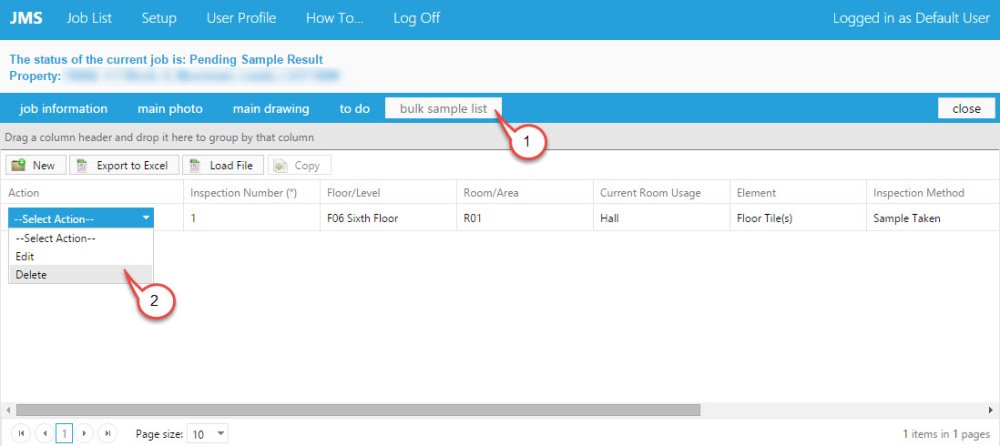The image depicts a website interface set against a white background. In the upper left corner, a light blue banner displays the company name "JMS" in bold white text. Stretching from left to right across the banner is the menu, featuring options such as "Job List", "Set Up", "User Profile", "How To", and "Log Off". In the upper right corner, it indicates the user is "Logged in as: Default User."

Beneath, a white banner reads in blue text: "The status of the current job is pending sample results." Below this is another blue banner with white text, listing sections from left to right: "Job Information", "Main Photo", "Main Drawing", and "To Do." Adjacent to this is a white box labeled "Bulk Sample List." To the right of the box, there's a white action button labeled "Close."